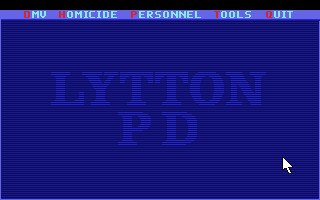This image is a screenshot of what seems to be the homepage of the Lytton Police Department's internal tool or database. The title "Lytton PD" is prominently displayed at the top in light blue text against a dark blue background. Just above this title, there's a black navigation bar with menu options including "DMV," "Homicide," "Personnel," "Tools," and "Quit," each written in very light blue letters with the initial letter highlighted in red. In the lower right portion of the image, a white arrow pointer, presumably a mouse cursor, is visible. The layout indicates an interface designed for administrative or operational use within the police department.